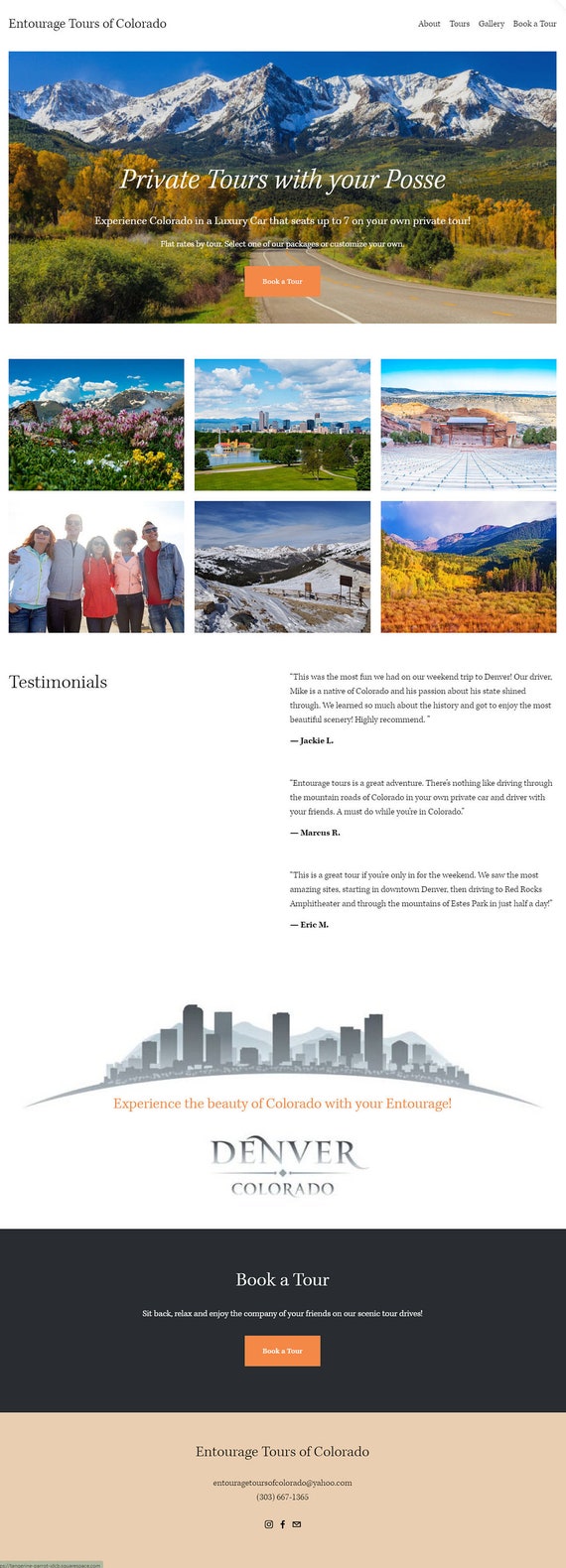The image appears to be a screenshot of a tourism website for Entourage Tours of Colorado. The layout is visually appealing, designed to attract people interested in exploring Colorado's scenic landscapes.

At the top right corner, the navigation menu displays prominent categories: "Book a Tour," "Gallery," "About," and "Tours." On the top left, the website proudly showcases its name, "Entourage Tours of Colorado."

Directly below the website's title is a captivating image depicting majestic mountains, verdant trees, and a winding road, encapsulating the spirit of adventure. Superimposed on this image are the words "Private Tours with your Posse," suggesting an exclusive and intimate tour experience.

Further down, a brief description reads, "Experience Colorado in a luxury car that seats up to seven on your own private tour," highlighting the comfort and exclusivity offered. Below the description, an orange button labeled "Book a Tour" invites users to take the next step in planning their adventure.

The lower section of the page features a gallery arranged in two rows of three images each. The top row includes:
1. A vibrant picture of flowers.
2. A serene grassy area with a tranquil lake.
3. An intriguing stone-filled landscape.

The bottom row includes:
1. A group photo of five smiling people.
2. Snow-capped mountains exhibiting the rugged beauty of Colorado.
3. A sprawling forest showcasing an array of yellow, red, and green foliage.

At the very bottom center of the image, the website reiterates its name, "Entourage Tours of Colorado," reinforcing brand identity.

This detailed layout effectively conveys the allure and customizable nature of the tours offered, inviting visitors to explore Colorado in luxury and style.